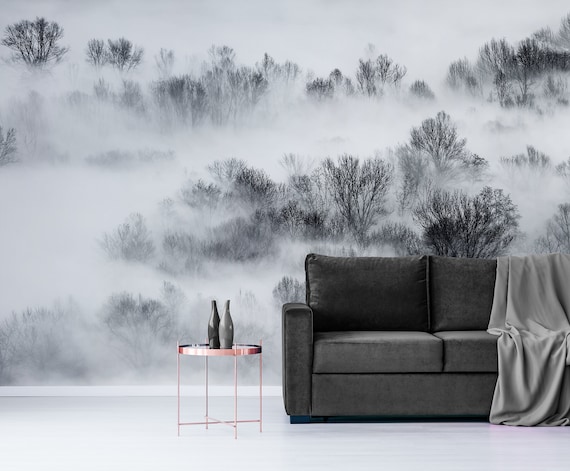The image depicts a plain, minimalist room captured in black and white. Dominating the right side is a dark gray or black couch adorned with a lighter gray blanket draped over the middle, flowing down to pool on the floor. Adjacent to this couch is a round, bronze-colored metal end table with a glass top and distinctive four legs with a crossbar. On this table sit two uncapped, grayish wine bottles. The flooring is a simple grayish-white, transitioning to a white baseboard that runs along the room's perimeter. The back wall features an intricate black and white mural, portraying a foggy outdoor scene with various levels of dark bushes and trees, creating a sense of depth and mystery. This wallpaper extends seamlessly across the wall, enveloping the room in a misty, dreamlike ambiance.